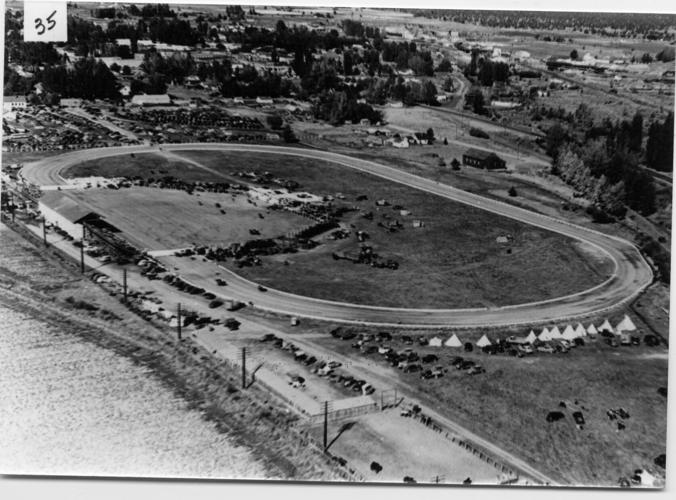This black and white aerial photograph, taken outdoors under natural light, prominently features a large oval racetrack, likely designed for cars. The image is primarily square-shaped with a subtle gray border along the top and bottom edges. In the upper left corner, there is an artificially added white square with the hand-drawn number "35." Around the racetrack, which stretches over a vast area, multiple vehicles, including pickups and cars, are parked near white teepee-like structures and tents. Sparse housing and numerous trees dot the surrounding landscape, which transitions into open land rather than a dense urban setting. Visible power poles are situated to the left of the track, and there is also a building near the track for spectators.